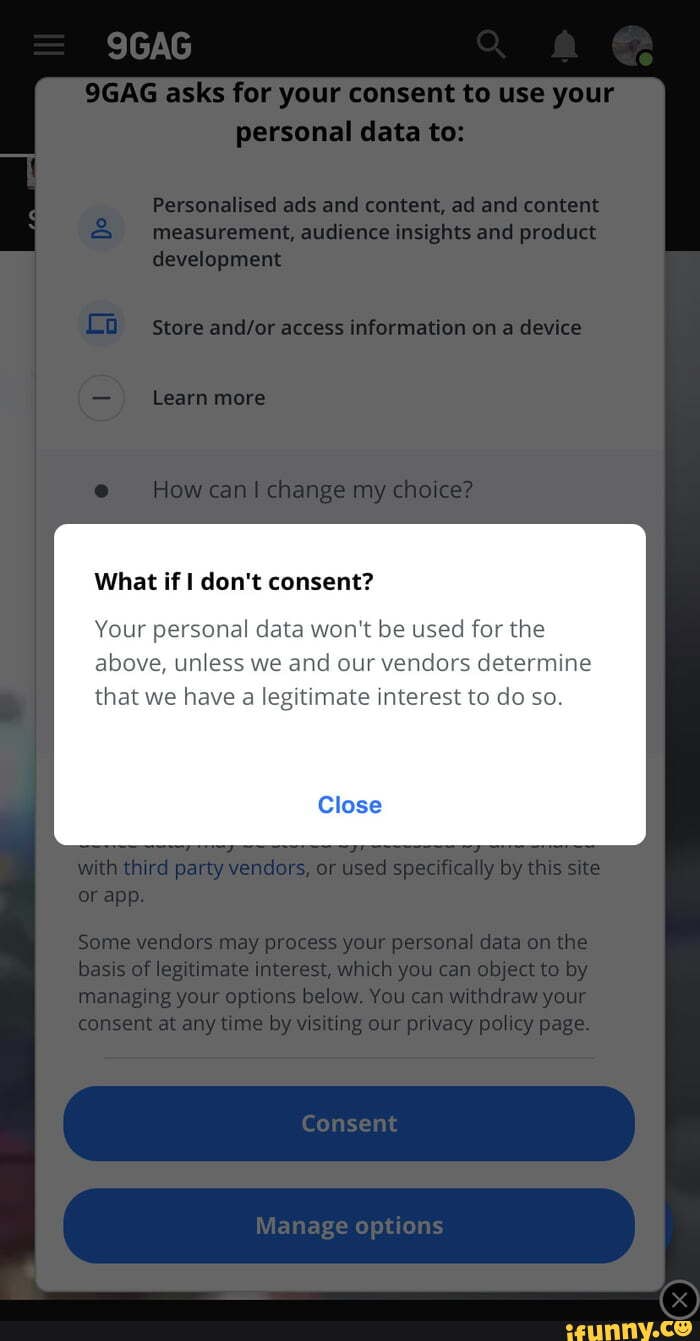The image is a screenshot from a cell phone, displaying a notification over a grayed-out background screen. The background is slightly opaque, making it difficult to discern the details clearly. In the foreground, there is a white rectangular notification box with curved edges, containing a message which reads: "What if I don't consent?" Below this, additional text states that "your personal data won't be used for the above unless we and our vendors determine that we have a legitimate interest to do so." 

At the very bottom of the notification, there is an option labeled "Close." 

Faintly visible in the background, the website 9GAG is requesting consent for the use of personal data. Accompanying this message are three small blue icons representing the different categories of data use, with explanatory text nearby printed in black. The overall tone of the image conveys a concern for privacy and data consent, marked by the clear visibility of the consent query against the blurred backdrop.